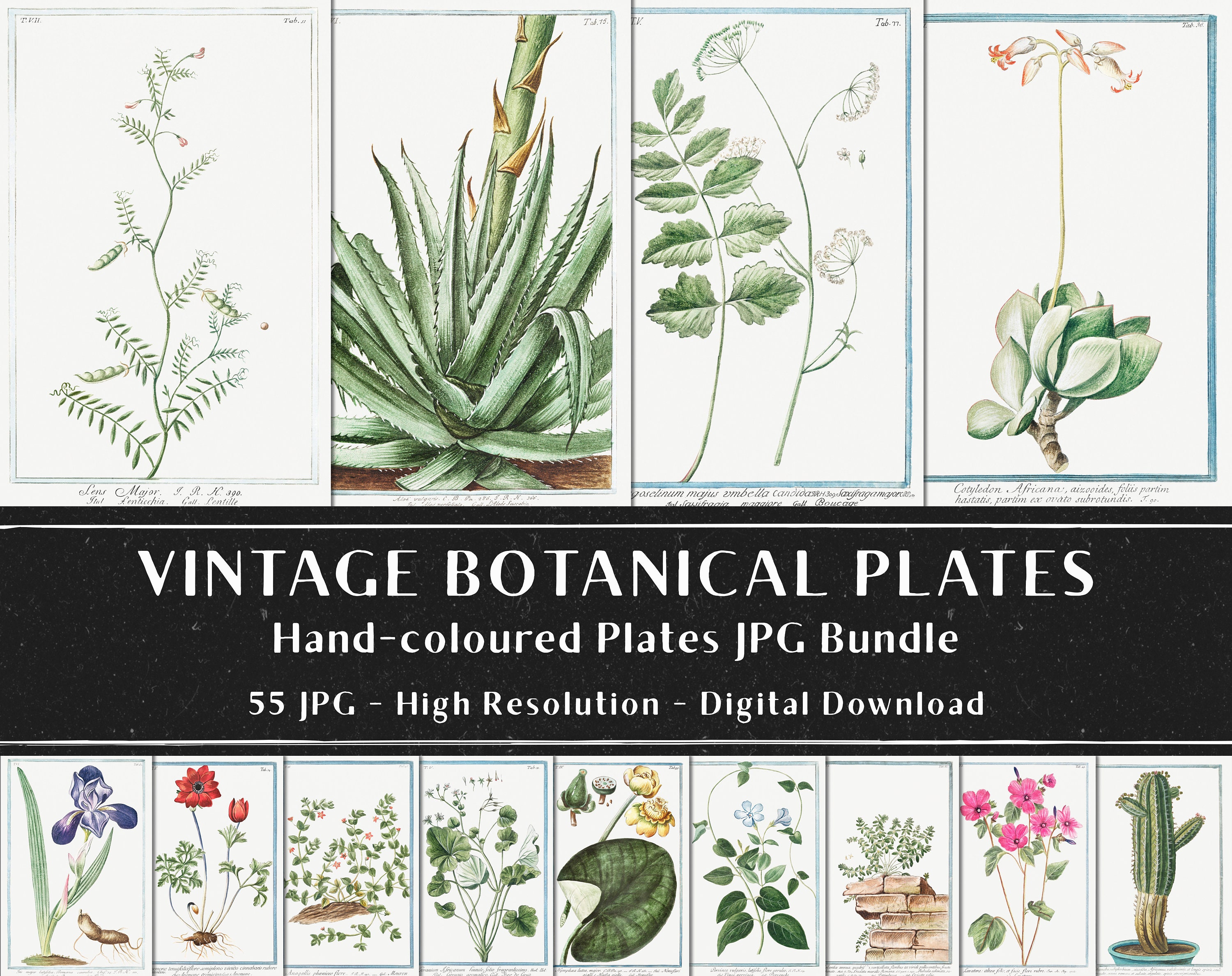This image is an advertisement for a digital download collection of vintage botanical plates. The composition features an array of highly detailed botanical illustrations divided into two main sections, with a black banner in the center. The banner includes white text reading "Vintage Botanical Plates" followed by "Hand Colored Plates JPEG Bundle" and "55 JPEG High Resolution Digital Download" in smaller font below. 

In the top section, there are four vertical botanical illustrations: 
1. On the left, a wispy green plant with a curvy stem running from bottom to top.
2. To its right, a sharp-leaved green plant with a green stalk topped by brown triangular shapes.
3. Next, two plants; one with a thin green stem and green leaves, and the other, taller with a thin stem and buds at various angles.
4. The far right shows a brown stick-like plant with green leaves, yellow tendrils climbing to the top, adorned with white and orange flowers.

The bottom section contains nine additional vertical plates:
1. A purple flower on the left.
2. Beside it, a red flower resembling a poppy.
3. Next, green leaves.
4. A crown-shaped green plant.
5. A large green leaf.
6. A small plant with green leaves and blue flowers.
7. A plant growing out of brown bricks with green leaves.
8. Pink flowers with green leaves.
9. A tall cactus with buds extending from it.

Overall, the image showcases a diverse range of plants including cacti, succulents, flowers, and small weeds, all rendered with vibrant colors and meticulous detail.